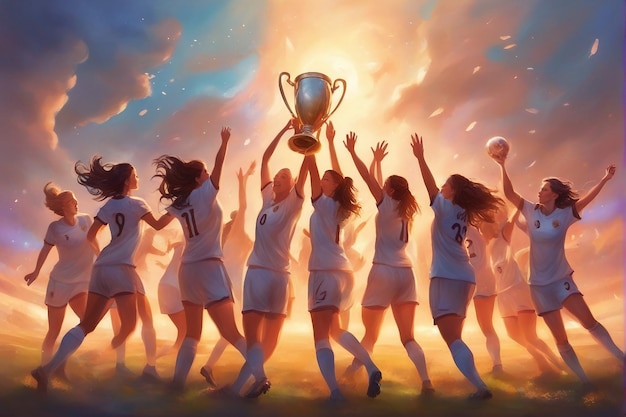The image is a dynamic illustration of a victorious team of female soccer players celebrating a recent win. The girls are dressed in white knee-length socks, white shorts, and uniform polo shirts with blue trims on the edges of their sleeves and shorts. Dark-colored numbers can be seen on some of their uniforms, with 11, 9, 8, 6, and 2 visible. Two players in the middle proudly hoist a large trophy above their heads, while most of the other players raise their arms in jubilation. One girl on the right stands out, holding a soccer ball in her right hand as she joins in the celebration. The background features a surreal sky with blue patches and clouds, blending into a greenish-yellow surface that suggests an explosion of light, adding to the dynamic energy of the scene. This vivid combination of intricate details and triumphant expressions encapsulates the team's elation and sense of achievement.